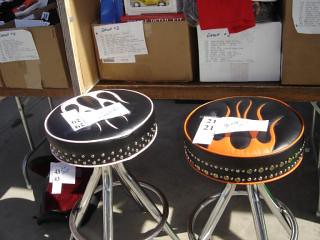The image depicts two chrome-legged bar stools positioned outdoors on asphalt pavement. Each stool features a circular black leather cushion embellished with a distinctive flame design: the left stool displays white flames, while the right showcases a combination of red, yellow, and orange flames. Both stools have white stickers on them, with the leg supporting footrests encircling the legs. In the background, there's a board against the wall, covered in variously colored papers—predominantly white, red, blue, and black—fastened with thumbtacks. Additionally, there is a dark brown table nearby, laden with white and brown boxes bearing white stickers. Underneath the right stool, an indistinguishable black object with red markings can be seen.